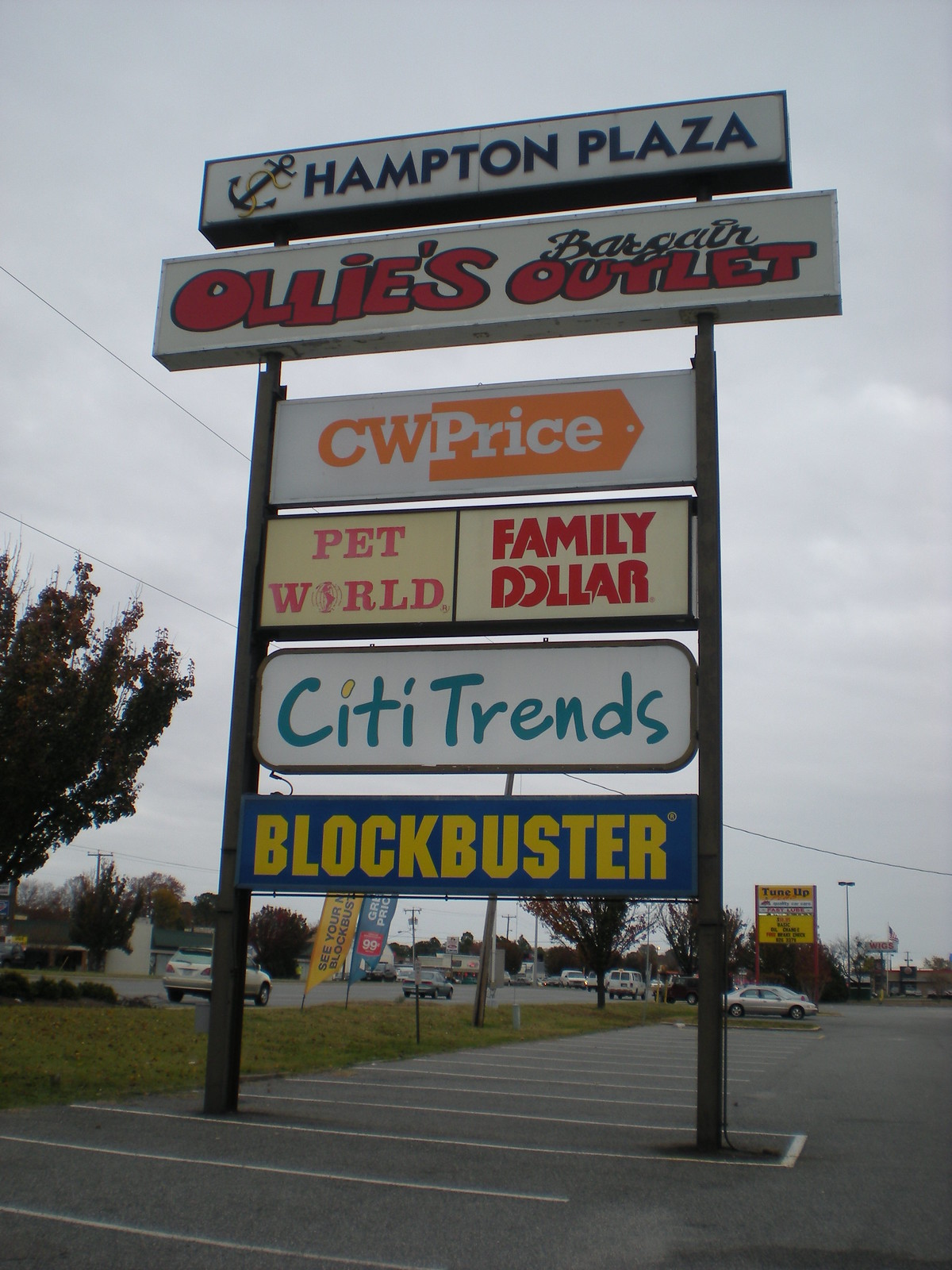The image depicts a large sign at the edge of a mall parking lot, featuring advertisements for various stores within the Hamilton Plaza. The sign is supported by two substantial metal poles and is composed of six separate panels. At the very top, the largest sign reads "Hamilton Plaza" accompanied by an anchor symbol. Below it, in descending order, the signs list:

1. Ollie's Bargain Outlet
2. CW Price
3. Pet World (left) and Family Dollar (right) — both smaller signs positioned side by side
4. City Trends
5. Blockbuster

In the background, cars are visible driving by, indicating a bustling area. A secondary, smaller sign promoting a car tune-up service is also noticeable in the distance. To the left of the sign, there is a tree, and the expansive, gray sky dominates much of the background, giving the scene a somewhat overcast ambiance.